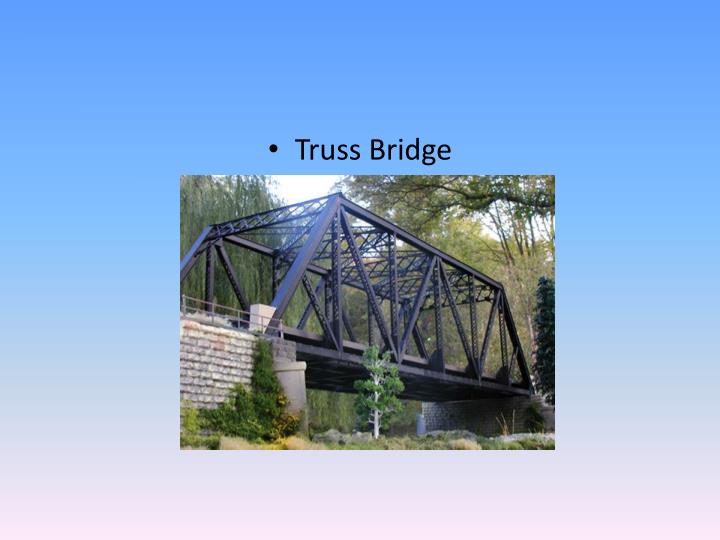The image appears to be a slide from a PowerPoint presentation, characterized by a gradient background transitioning from dark blue at the top through light blue and white, to a pale light pink at the bottom. At the center of the slide is a rectangular photo of a well-maintained truss bridge constructed from black iron or steel. The bridge is anchored on either side by brick walls and surrounded by abundant vegetation, including tall trees with green leaves, grass, and shrubberies. The backdrop behind the bridge emphasizes a bright, slightly cloudy sky with sunlight filtering through the trees. Above the image, in a black font, there's a title that reads ". Truss Bridge."